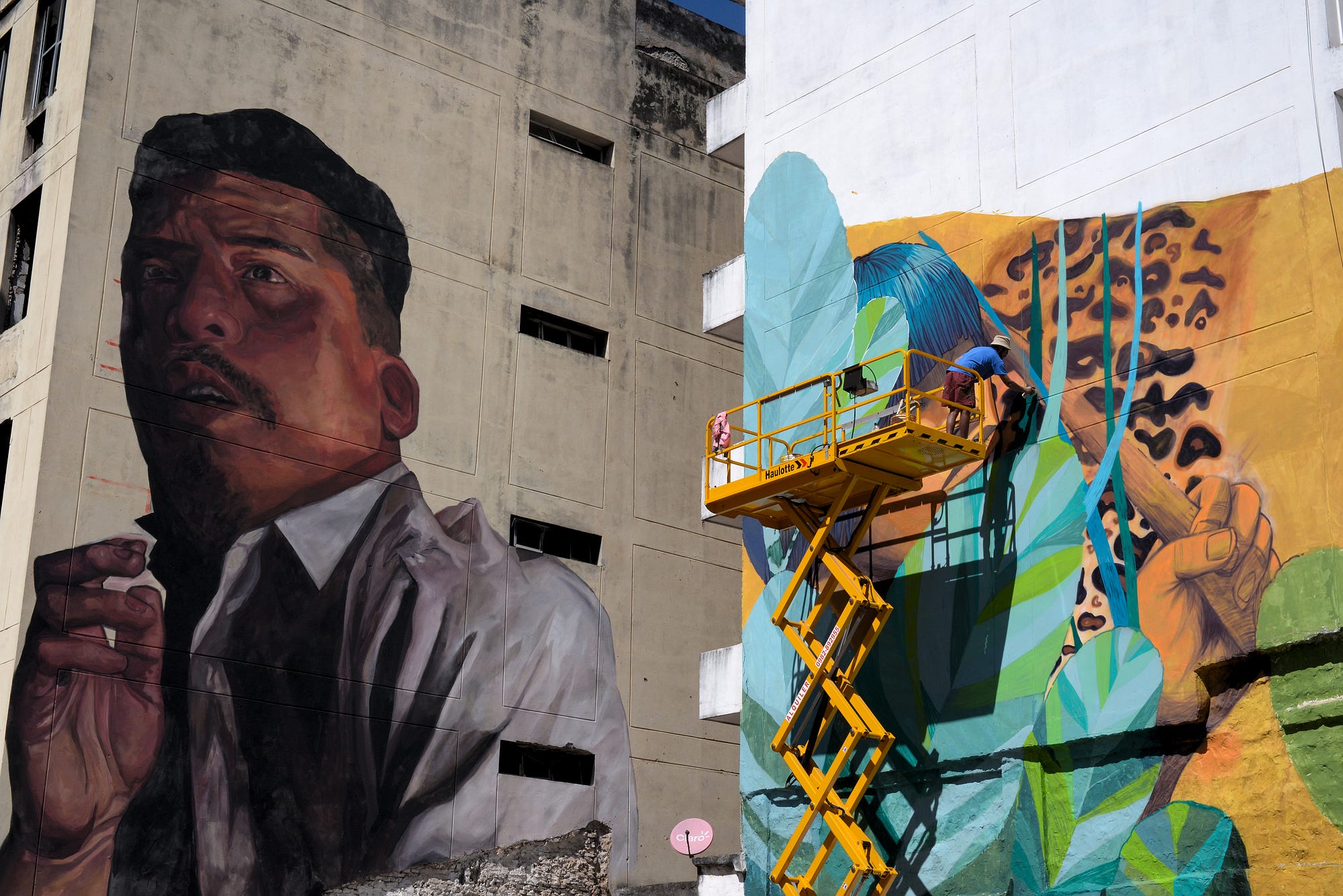This color photograph captures a vibrant street art scene on the sides of two adjacent buildings beneath a clear, cloudless blue sky. On the left, a gray building features a detailed mural of a man with dark, grayish-brown hair, a beard, mustache, and brown eyes. He wears a black hat, a gray over-shirt, and a black undershirt. The windows of this building are blackish, contrasted by the striking white collars of the man's shirt. 

The building on the right is white with several balconies protruding from its side. One of these balconies has a gray satellite dish with unreadable white text. A yellow scaffold is positioned against this building, where an artist, dressed in a blue t-shirt and cap, actively works on a colorful mural. This mural is partially completed and features various elements: a hand holding a stick, leaves in shades of blue and green, and a segment of tan, black, and brown cheetah print. The painter is creating the artwork while standing on the scaffold. The dynamic scene is enhanced by the intricate details of the mural and the serene gap of blue sky visible between the buildings.